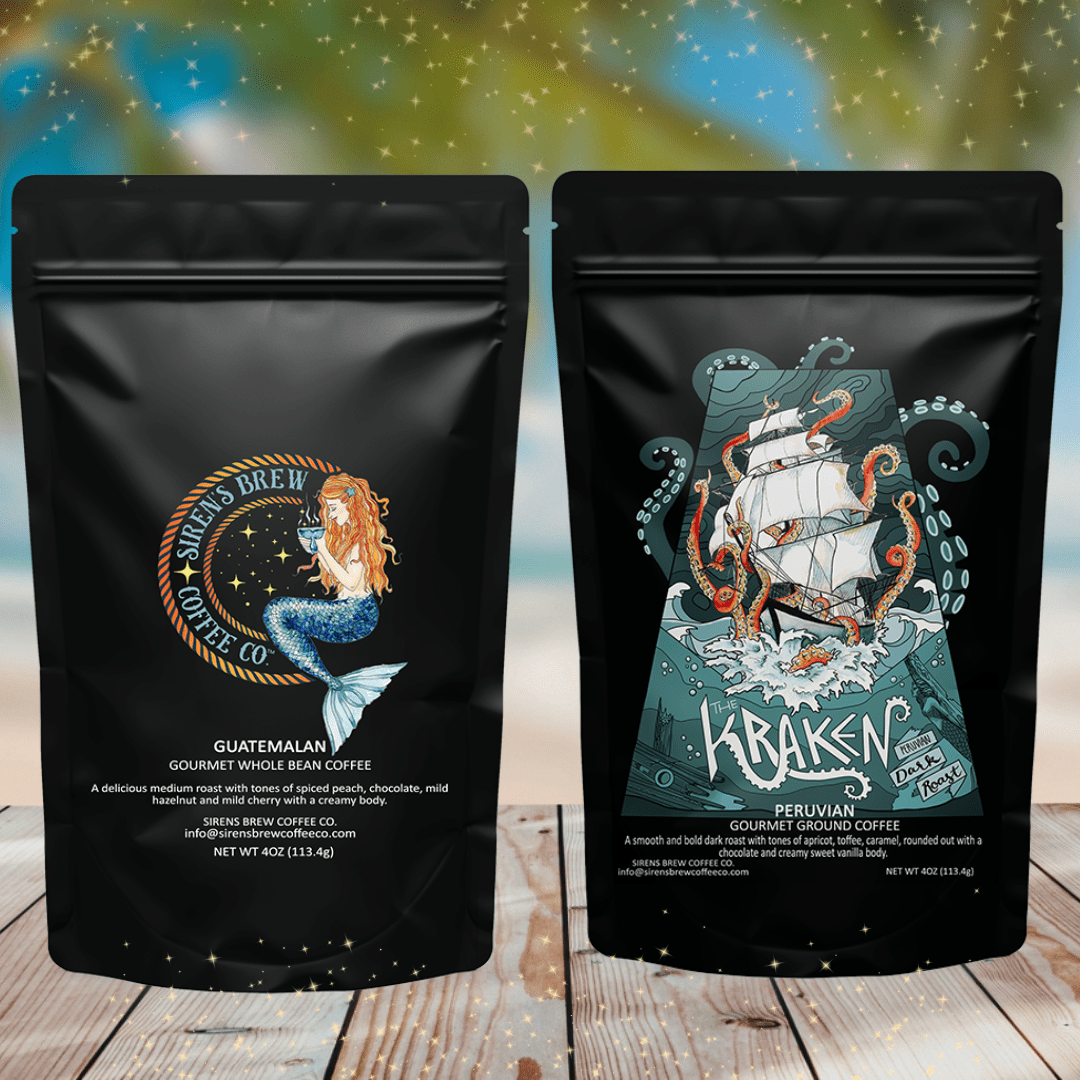This is a detailed photograph of two black coffee packages sitting on a wood grain table, possibly a picnic table, with a greenish, starry, computer-generated background. The package on the right features an ominous illustration of a ship being attacked by a massive Kraken, with its tentacles wrapping around the vessel. This package is labeled "Peruvian Gourmet Ground Coffee" in white text, and underneath, in smaller, less legible white text, there are likely details about the flavor, net weight, and company contact information. This coffee is identified as a dark roast. 

The package on the left showcases a mermaid with long red hair, likely sipping coffee from a cup, under the label "Sirens Brew Coffee Company." It prominently states "Guatemalan Gourmet Whole Bean Coffee" in white text. Below, there's a detailed flavor description mentioning a delicious medium roast with tones of spiced peach, chocolate, mild hazelnut, and mild cherry, boasting a creamy body. This package also provides the net weight of 4 ounces and possibly additional coffee-related information in smaller, legible text. 

Both packages are positioned prominently on the table, emphasizing their detailed and vibrant imagery against the artistic backdrop.